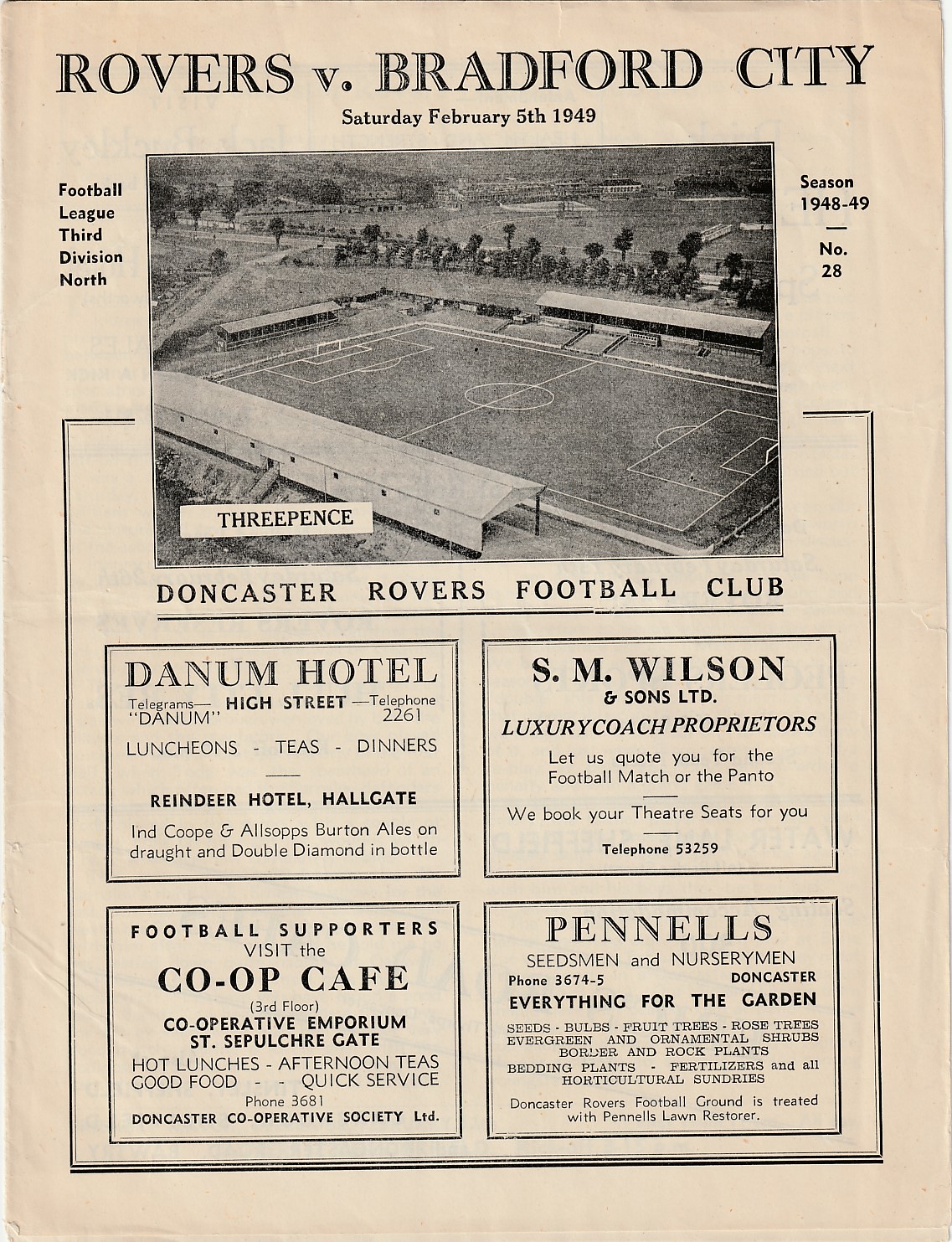This image depicts a vintage advertisement from the 1948-1949 season for a football match between Doncaster Rovers and Bradford City. The ad is printed in black on an aging off-white paper and features bold text at the top that reads "Rovers versus Bradford City," with the match scheduled for Saturday, February 5th, 1949. Below, in smaller text, it notes "Football League Third Division North," alongside the season details, "1948-1949,” and the designation “number 28."

Central to the ad is a black-and-white photograph of a football pitch viewed from above, framed by stands on the left and right. The inset in the photo specifies an entry fee of three pence. The lower section of the advertisement features a black square containing four sponsor advertisements: Danum Hotel located on High Street, S.M. Wilson’s Luxury Coach services, Co-op Cafe, and Pennell’s store. The image and text collectively evoke a nostalgic feel of a bygone era in English football history, prominently showcasing the essence of Doncaster Rovers Football Club’s promotional efforts in mid-20th century England.